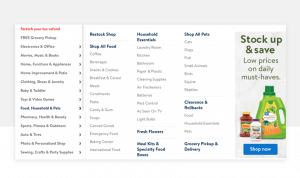The image displays a promotional flyer for grocery products. On the right-hand side, there is a bolded, black text that reads "Stock Up and Save" inside a rectangular box, emphasizing the savings. Below it, the text states "low prices on daily must-haves," although the image resolution makes it difficult to discern specific items. 

On the left-hand side, a green bottle resembling laundry detergent is visible, along with a jar of spaghetti sauce adjacent to it. Between these items, there is a white area with an unidentified object. At the bottom, there is a rectangular blue button labeled "Shop Now," suggesting a call to action for the viewer.

The left-hand side of the flyer features a white section with red text at the top, which is organized into multiple rows extending to the bottom. Each row ends with unspecified content. Additionally, there are three columns with several blue-highlighted areas containing additional rows, although some columns are missing content. The overall design indicates various grocery deals and calls for shoppers to take advantage of savings.